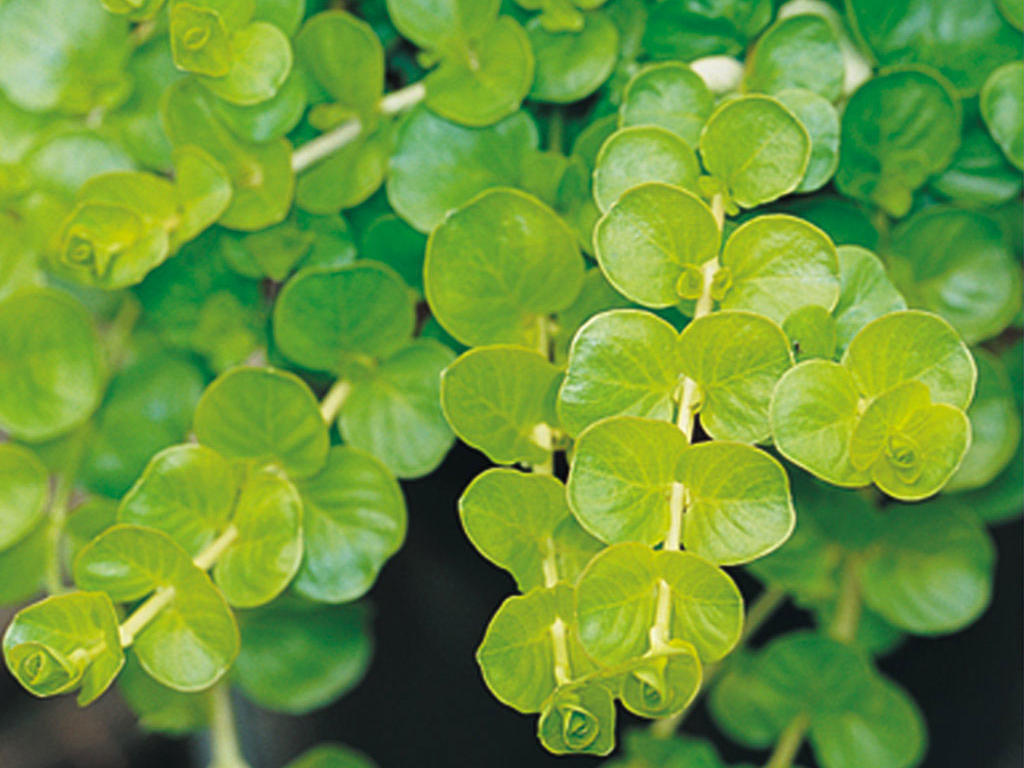The image, in landscape orientation, is a close-up of a vibrant eucalyptus plant, illuminated by bright lighting that accentuates its lush green foliage. The plant features several long, white stems with round, almost heart-shaped leaves arranged in pairs on either side of the stem, giving an impression of symmetry and balance. The tips of the stems showcase new growth, often curling elegantly like a rose. In the foreground, about seven or eight stems stand out sharply against the dark, almost black background, which is only faintly visible through the dense greenery. The background contains additional stems of the same plant, slightly out of focus, creating a sense of depth and suggesting that the plant is either a large bush, tree, or possibly held in a vase. The overall appearance of the plant is healthy and mature, exuding a fragrant and robust feel that almost allows one to sense its aroma through the image.